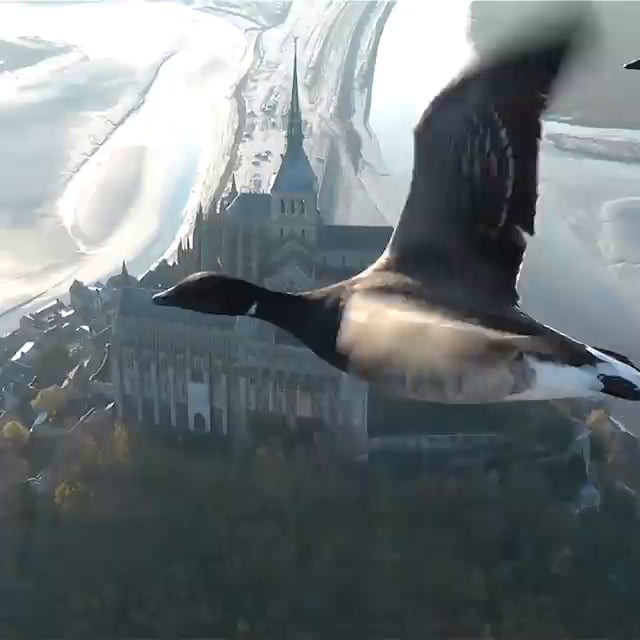This photograph captures a mallard duck in mid-flight, prominently positioned against a somewhat blurry background that includes a large, elaborate castle enveloped by a dense collection of green trees. The castle, anchored by a tall steeple, stands at the center of the scene with its intricate architecture obscured partly by the flying bird. The skies, filled with clouds, add depth to the scene, and there appears to be a hint of an ocean or some other ambiguous landscape feature in the distance. The duck itself, with its black head, black beak, and black neck leading to a white-striped body, commands attention in the foreground, its wings spread wide as it glides through the air. Interestingly, another duck's beak intrudes into the frame from the top right, adding a touch of surprise and dynamic movement. The overall composition suggests either a unique photographic moment or a digitally manipulated image, combining natural and fantastical elements.